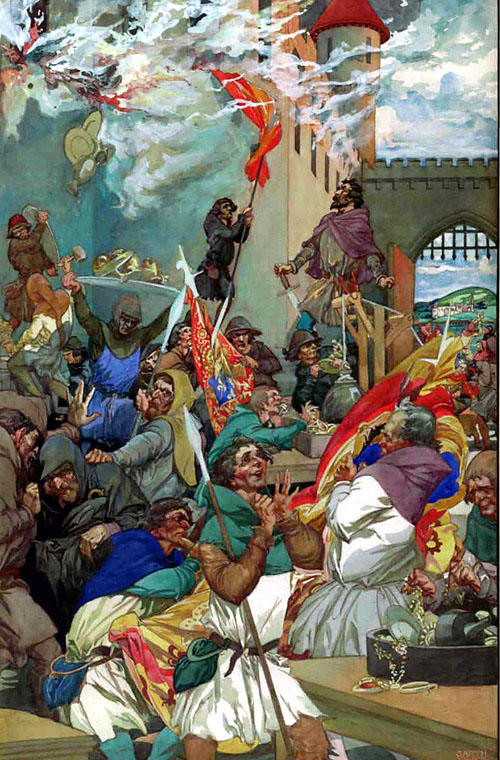This detailed painting illustrates a bustling medieval scene set within the courtyard of a castle. Amidst the lively hullabaloo, approximately 20 to 30 figures in colorful peasant garb and a few chain-armored soldiers create a vivid tableau of a castle raid. Smoke billows from the upper parts of the castle, suggesting gunshots or some form of conflict, while flags and spears are prominently displayed. The scene is chaotic, with people carrying treasures such as golden goblets on flat plates, and others involved in various forms of commotion, including punching and fighting, reminiscent of a civilian protest. An open gate on the right reveals green hills in the background, adding depth to the tumultuous atmosphere. A man at the bottom of the painting appears to revel in the disorder, his expression one of sheer delight amidst the mayhem. Tables scattered throughout the courtyard bear all sorts of treasures and plates, enhancing the rich, chaotic ambiance of this medieval spectacle.